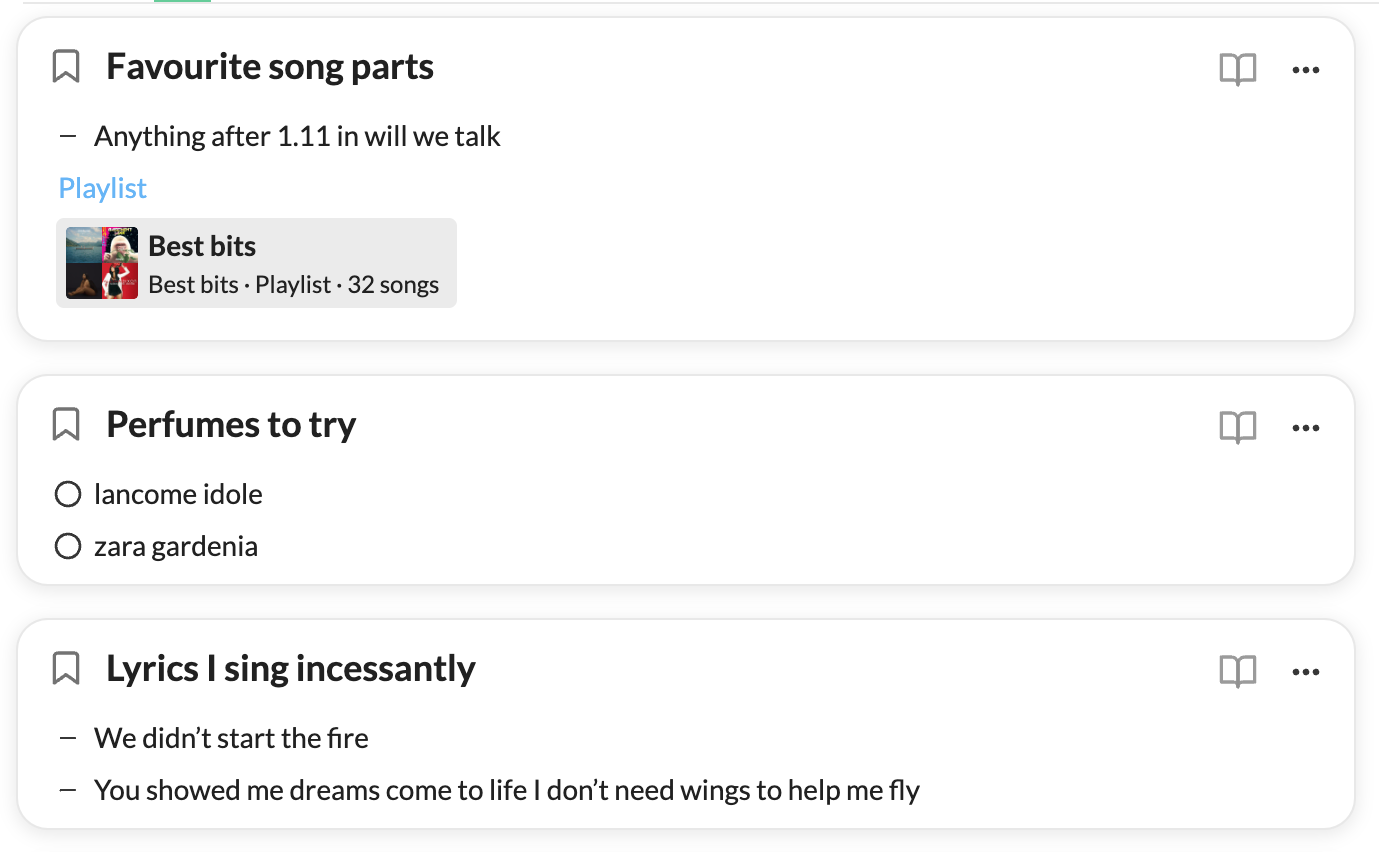This image displays a music playlist screen composed of three main sections, each designed with specific icons and text arrangements.

**Top Section:**
- **Icons:** 
    - Bookmark icon at the top left
    - Book icon at the top right
    - Three-dot menu icon to the far right
- **Text:**
    - "Favorite Song Parts" in bold at the top
    - Below that, a dash followed by "Anything after 1:11 in we will talk"
    - The word "Playlist" highlighted in blue
    - A small inner box with the text "Best Bits · best bits · playlist · 32 songs"
    - Collage of four album covers

**Middle Section:**
- **Icons:**
    - Bookmark icon at the top left
    - Book icon at the top right
    - Three-dot menu icon to the far right
- **Text:**
    - "Perfumes to Try" at the top
    - Two circles with text inside:
        - The first circle: "Young Comb I Dole"
        - The second circle: "Zara Gardenia"

**Bottom Section:**
- **Icons:**
    - Bookmark icon at the top left
    - Book icon at the top right
    - Three-dot menu icon to the far right
- **Text:**
    - "Lyrics I Sing Incessantly"
    - Below that, a dash followed by specific lyrics:
        - "We didn't start the fire"
        - "You showed me dreams come to life, I don't need wings to help me fly"
    - Album covers are somewhat unclear but identifiable:
        - Top left: Appears to feature a river valley
        - Top right: Resembles an artwork of Lady Gaga
        - Bottom right: Red background with a singer
        - Bottom left: Black background with a golden singer

This detailed breakdown of the playlist screen perfectly captures the structure and content of each section, providing a comprehensive understanding of the visual and textual elements.